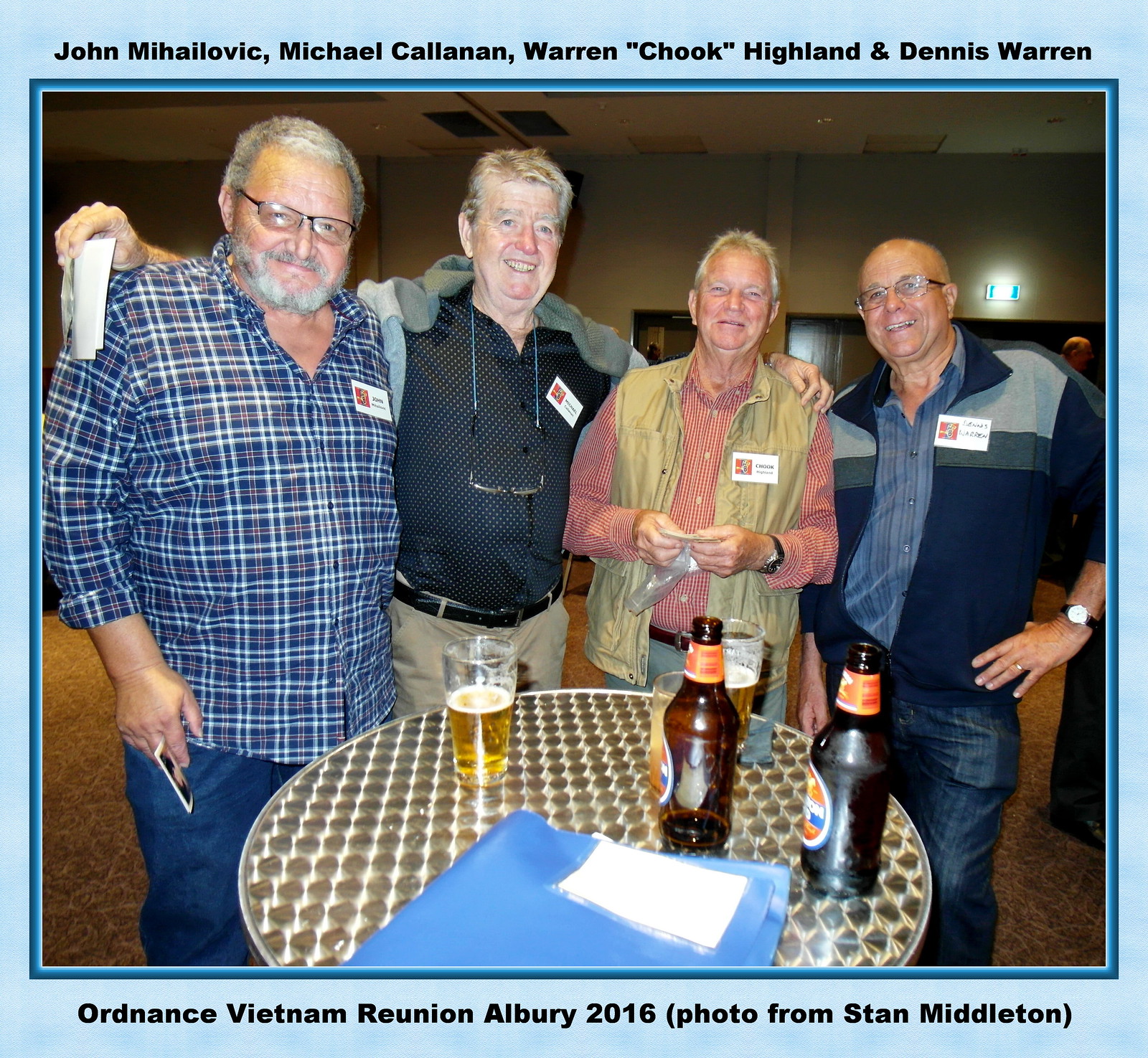In this vibrant photograph with a light blue border, four older gentlemen, likely in their 60s to 80s, stand arm in arm behind a round table adorned with pint glasses and bottles of beer. The men are smiling warmly at the camera, exuding camaraderie and joy. Each man wears a collared shirt and name badge on the left side of his chest. Notably, two of them sport glasses, and one has a beard. The image captures the spirit of a reunion, underlined by the black text at the top and bottom of the photo, which reads: "John Mihaljevic, Michael Kalanan, Warren 'Chook' Hyland, and Dennis Warren" and "Ordnance Vietnam Reunion, Albury 2016, photo from Stan Middleton." The setting appears to be an indoor event celebrating their shared history as Vietnam veterans.